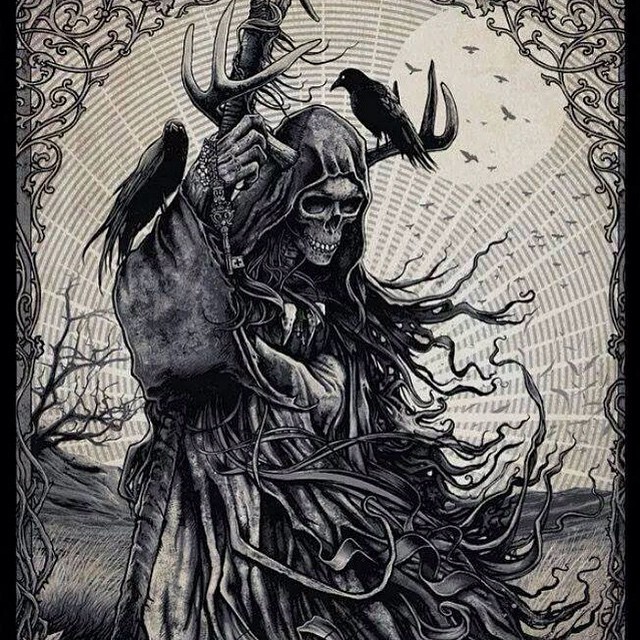This intricate black, white, and gray ink drawing depicts a dark, ominous figure resembling the Grim Reaper. The skeletal figure, clad in a tattered, hooded robe, stands with rags and ribbons of material flowing around it. From its right hand, a wooden staff entwined with an elk horn extends downward, accompanied by a key dangling from it. Two crows perch on the figure – one on the antler and the other on its arm. The background features a large, circular moon with the silhouettes of birds or bats flying across it. Surrounding the composition, delicate fretwork and scroll-like decorations intertwine with gnarly trees at the bottom; particularly notable is a twisted tree on the left that seems to reach out and touch the skeletal figure, enhancing the eerie and foreboding atmosphere of the piece.